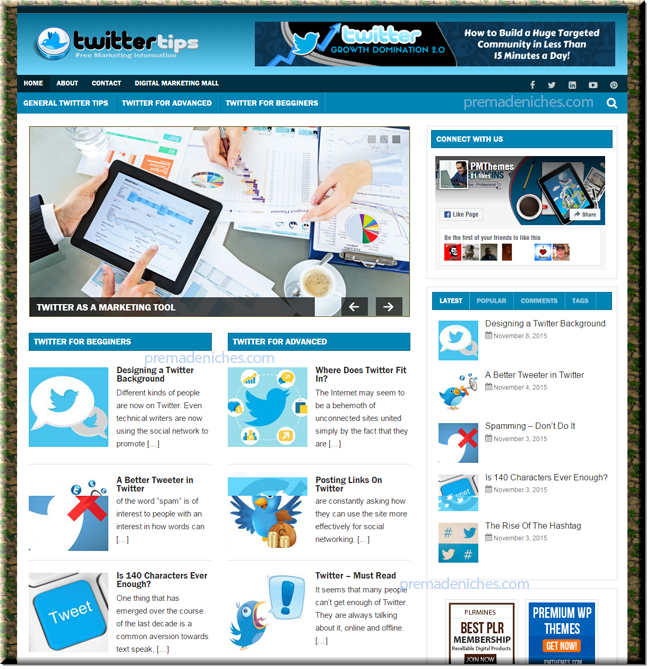The image is a screenshot of a webpage titled "Twitter Tips." At the top of the page, next to the bold black text "Twitter Tips," is the iconic Twitter bluebird emblem positioned within a circle. Directly beside this title, there's a light blue rectangle block featuring the Twitter bird logo and the word "Twitter" in light blue text. The description "Growth Domination 1.0: How to build a huge targeted community in less than 15 minutes a day" is prominently displayed beneath the title.

On the left-hand side of the webpage, navigational tabs labeled "Home," "About," "Contact," "Digital Marketing," and "Mall" are listed. Below these tabs, there's an organized section detailing general Twitter tips, as well as specific advice categorized for advanced users and beginners. 

Accompanying the text is an illustrative picture showing two sets of hands engaged in an activity. One person is holding a tablet horizontally in the bottom left corner and is pointing at the screen, while another person, seated opposite, holds a pen in their right hand. The interaction occurs on a gray table, which also holds a glass of water, a cup of coffee with a spoon on the saucer, and several papers displaying graphical information.

Further down the webpage, clickable items offer instructional content such as "Twitter for Beginners," and guidance on "Designing a Twitter Background." Each of these sections includes a brief description and distinct logo images for easy identification.